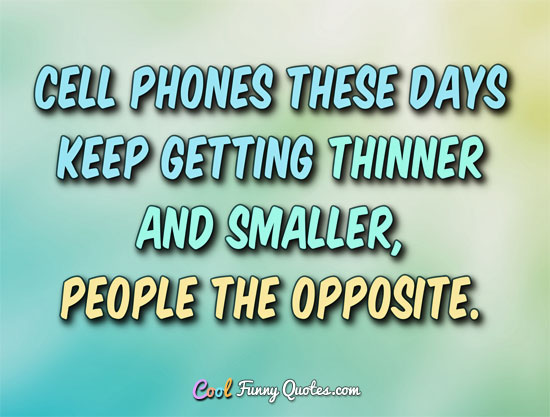The image features a poster with a lightly textured background transitioning from blue in the bottom left corner to lime green in the top right. In large, all-capital bubble letters, the poster humorously declares, "CELL PHONES THESE DAYS KEEP GETTING THINNER AND SMALLER, PEOPLE THE OPPOSITE." The phrase "CELL PHONES THESE DAYS KEEP GETTING" is in a light blue color, while "THINNER AND SMALLER" is in light green, and "PEOPLE THE OPPOSITE" stands out in yellow. At the bottom center of the poster, in small cursive white letters, it reads "funnyquotes.com." The word "COOL" above it is displayed in vibrant capital letters with each letter in a different color: C in magenta, O in pink, O in teal, and L in a light orange hue.